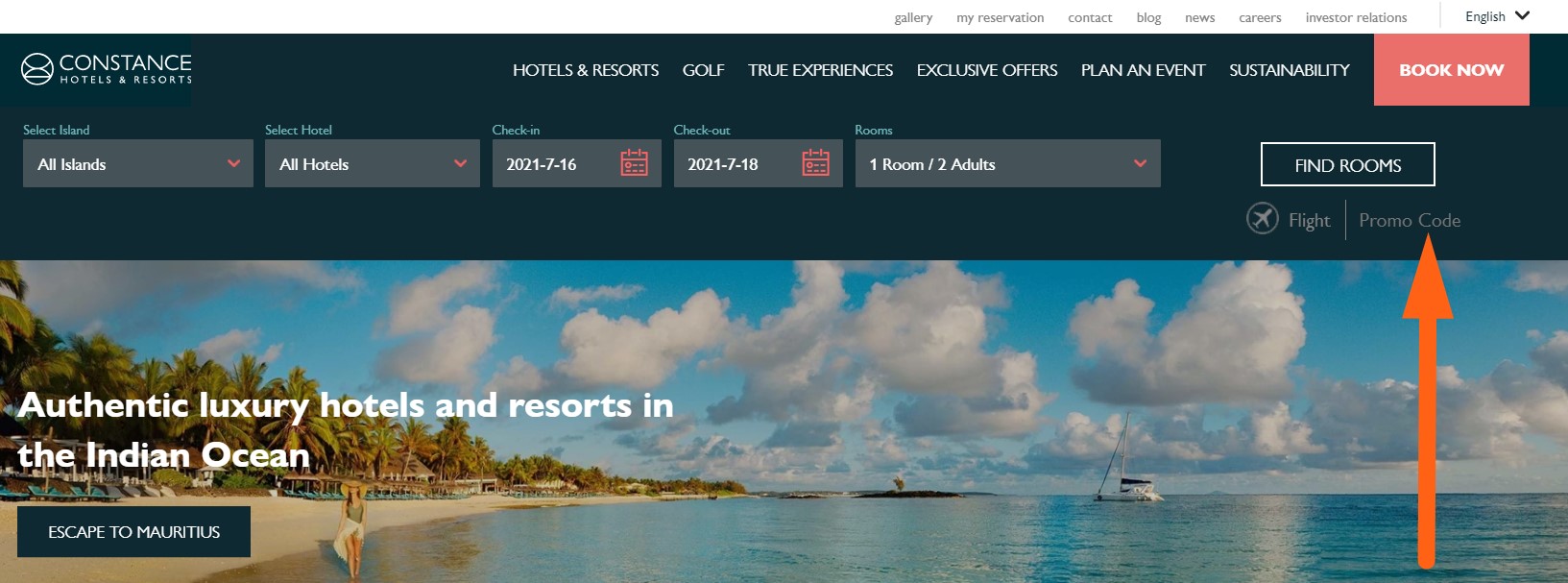The front page of a website for Constance Hotels and Resorts is presented in a horizontally cropped image, giving it a wide, expansive appearance. The top banner, coated in dark blue, prominently displays the brand logo on the top left, which features the text "Constance Hotels and Resorts" beside a circular emblem resembling two overlapping bridges. 

To the right of the logo, a navigation bar spans across the top, including sections labeled "Hotels and Resorts," "Golf," "True Experiences," "Exclusive Offers," "Plan Event," and "Sustainability," all in white text. On the top right, a red button with the text "Book Now" stands out.

Further up to the right side, there is another navigation area with a white background and black text. This section includes links to "Gallery," "My Reservations," "Contact," "Blog," "News," "Careers," "Investor Relations," and a dropdown menu for selecting the language, currently set to English.

Beneath these menus, options for booking are displayed, allowing users to select "Islands," "Hotel," "Check-In," "Check-Out," and "Rooms." A rectangular button with a dark blue background and white outline reads "Find Rooms" in white text. Below these booking options, there are fields for "Flight" and "Promo Code," the latter highlighted by an orange arrow pointing towards it from the bottom center-right of the image.

The lower portion of the image features a large banner showcasing a picturesque port-side beach scene. The right side shows a partly cloudy sky above a serene ocean, with a white boat floating nearby. On the left, a person strolls along the sandy beach, surrounded by lush tropical greenery and beach chairs.

In the bottom left of this banner, a dark blue rectangular button invites viewers to "Escape to Mauritius" in white text. Above this button, the banner reads, "Authentic Luxury Hotels and Resorts in the Indian Ocean." This scene encapsulates the enticing allure of a tropical getaway, promising a luxurious experience by the sea.